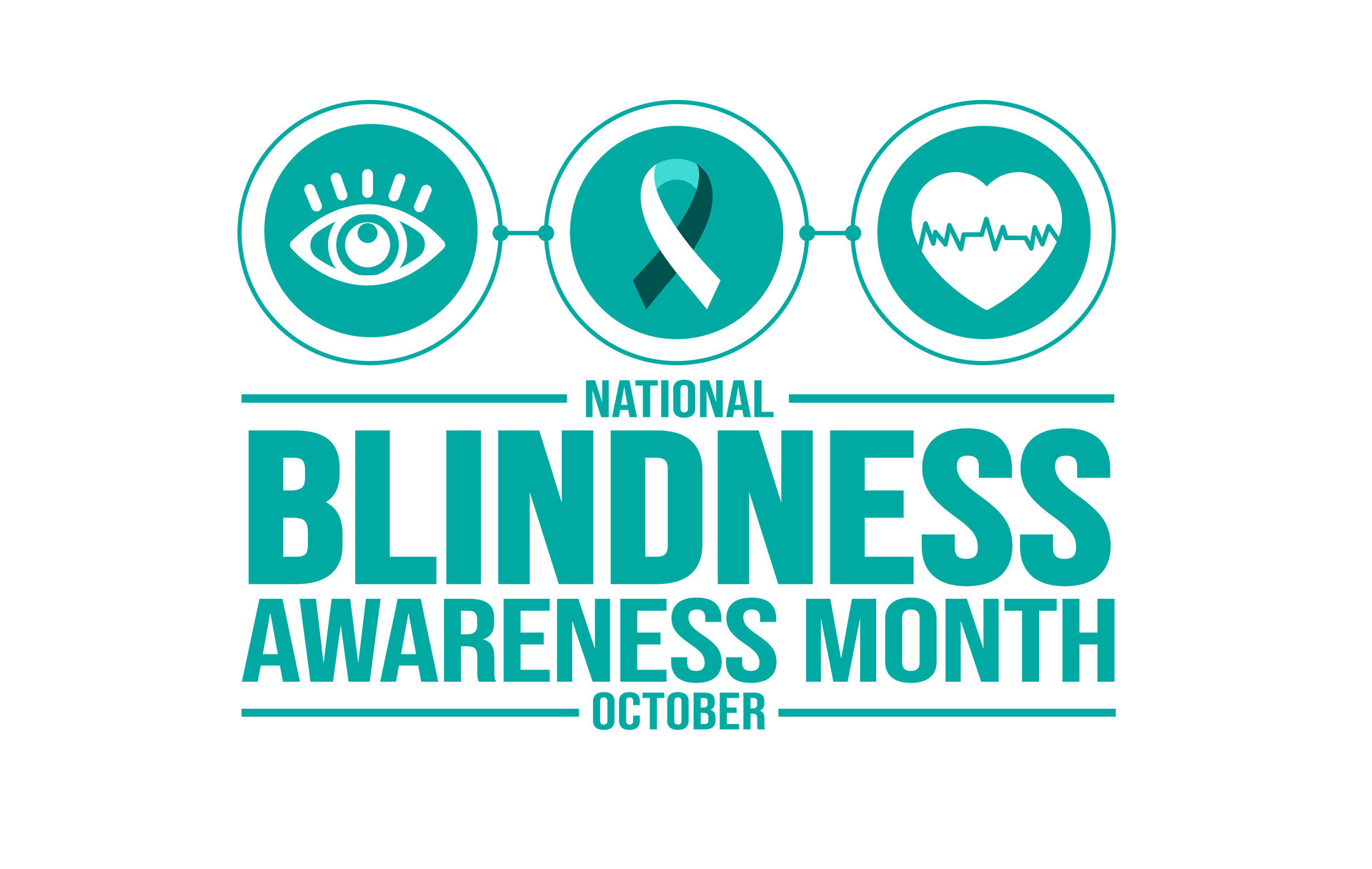The image is a graphic design on an all-white background, featuring three connected circles in a light blue-green color. Each circle is outlined with a thin white border and linked by small lines. The first circle on the left contains an outline of an eyeball with five dash-like lines above it, representing eyelashes. The middle circle features a ribbon similar to the breast cancer awareness ribbon, partially white and partially in a dark blue-green hue. The third circle on the right showcases a white heart with EKG-like pulse lines running across it. Below the circles, the text "NATIONAL BLINDNESS AWARENESS MONTH" is prominently displayed in capital letters of the same light blue-green color, with smaller text below stating "October." Additionally, thin blue-green border lines are placed on either side of the word "National" and the word "October".